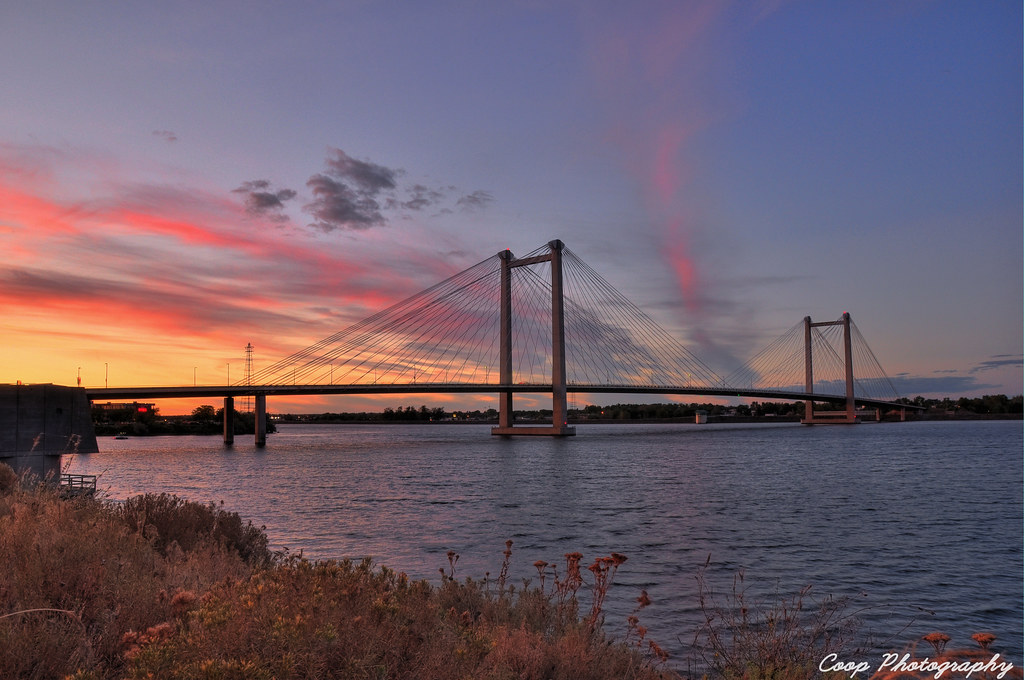The image features a large, serene body of water, likely a river or lake, under a subtly shifting evening sky. The sky at the top of the image transitions from light blue to a slightly darker hue on the left, with small gray clouds lower in the sky, tinged with pink and orange on the left side, likely reflecting the setting sun. Just below the horizon lies a strip of distant land spanning the width of the photo. Dominating the middle of the scene is a graceful bridge. This structure extends across the image from the middle left to the right, with a gentle arch descending toward the distant land. The bridge boasts two prominent sections, each featuring tall pillars connected by horizontal bars at both the top and water levels, with delicate wires draping down. On the left side, the foreground reveals a shoreline adorned with wildflowers and foliage that extends downward and right, sprinkling some flowers even off the bottom right edge. The water, illuminated by the sky, takes on both blue and pink hues, enhancing the tranquil ambiance. At the bottom right corner, the text "Coop Photography" is faintly inscribed.